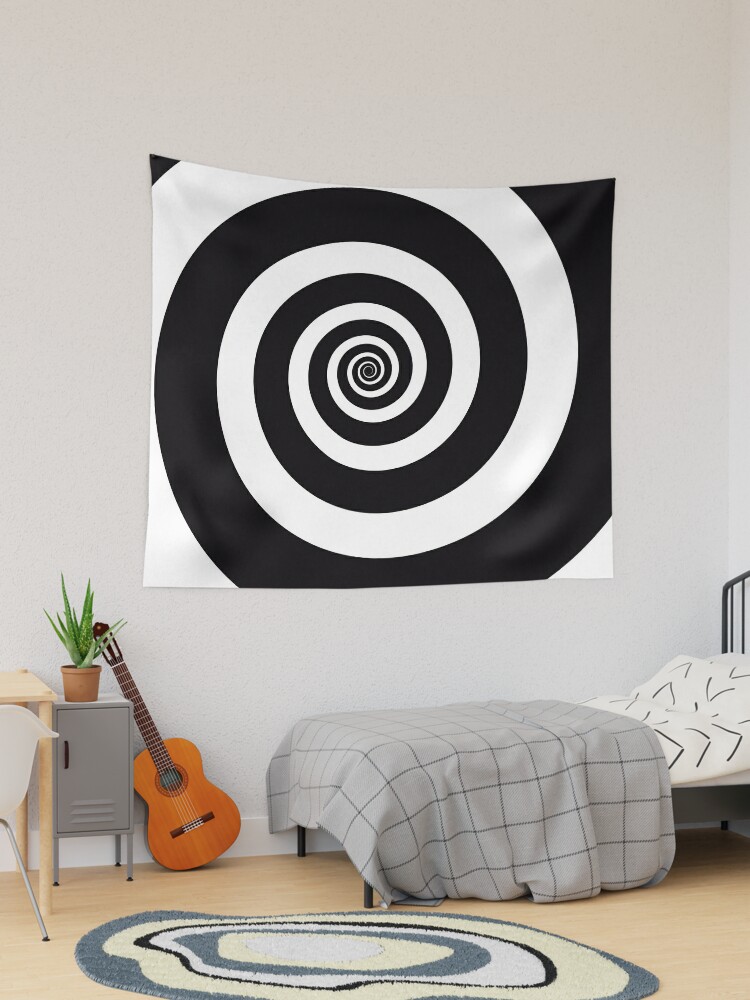The photograph showcases a cozy bedroom with white walls and light brown wood or linoleum flooring. Dominating the scene in one corner is a twin-size bed with a black metal frame, dressed in a gray plaid comforter and a white and black sheet set. Above the bed, a striking large square wall hanging featuring a black and white spiral design adds a touch of intrigue to the space.

At the foot of the bed rests an acoustic guitar, leaning against a gray metal locker-style end table. Atop this end table sits a brown flower pot housing a green aloe vera plant, adding a hint of nature to the room. Partially visible on the left edge of the frame is a pale wooden desk paired with a white plastic molded chair supported by metal legs.

The floor beneath the bed is adorned with an oval-shaped throw rug, boasting a swirly circular design in shades of gray, ivory, white, and black, harmonizing with the room’s understated, modern aesthetic.